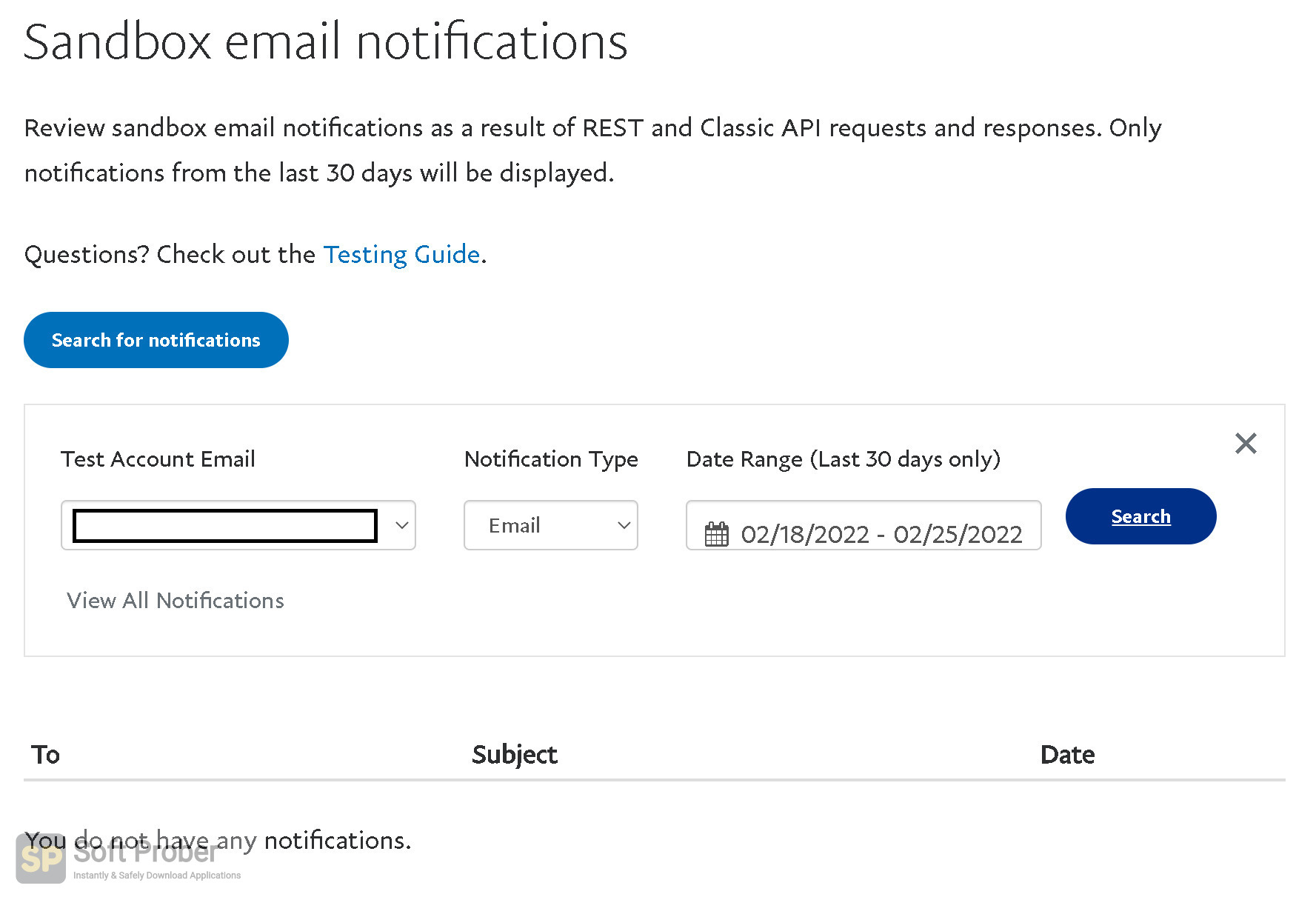The main colors of this interface are predominantly white and black, with occasional highlights of light blue. At the top left corner, there is a bold black header that reads "Sandbox Email Notifications." Directly below this header, in a smaller, darker black font, the text states: "Review sandbox email notifications as a result of" followed by "REST" in all capital letters and "and Classic API request and responses." Here, "Classic" is capitalized while "API" is fully capitalized. Further clarifying, it mentions, "Only notifications from the last 30 days will be displayed."

Continuing downward, there is additional text reading "Questions? Check out the testing guide," where "testing guide" is highlighted in light blue, indicating a clickable link. Below this snippet, a prominent blue oval button features the white text "Search for Notifications."

Beneath this button lies a white horizontal rectangular box outlined in light gray. The box is divided into sections. At the top left of the box, "Test Account Email" is indicated in black text, followed by "Notification Type" in the middle, and "Date Range (Last 30 days only)" to the right. At the far right end, there is a gray "X" mark, presumably for closing or dismissing the box. Each section is furnished with pull-down menus or search bars.

Under the "Notification Type" heading, a black text entry reads "Email." Below the "Date Range" heading, a specific date range is shown: "February 18th, 2022 to February 25th, 2022." Underneath the "Test Account Email" search bar, faint gray text displays "View all notifications."

Further down, the black text columns labeled "To," "Subject," and "Date" are lined up across the interface, awaiting user interaction or search results.

Overall, this well-organized and cleanly structured page is designed to help users review and search for specific sandbox email notifications effectively.